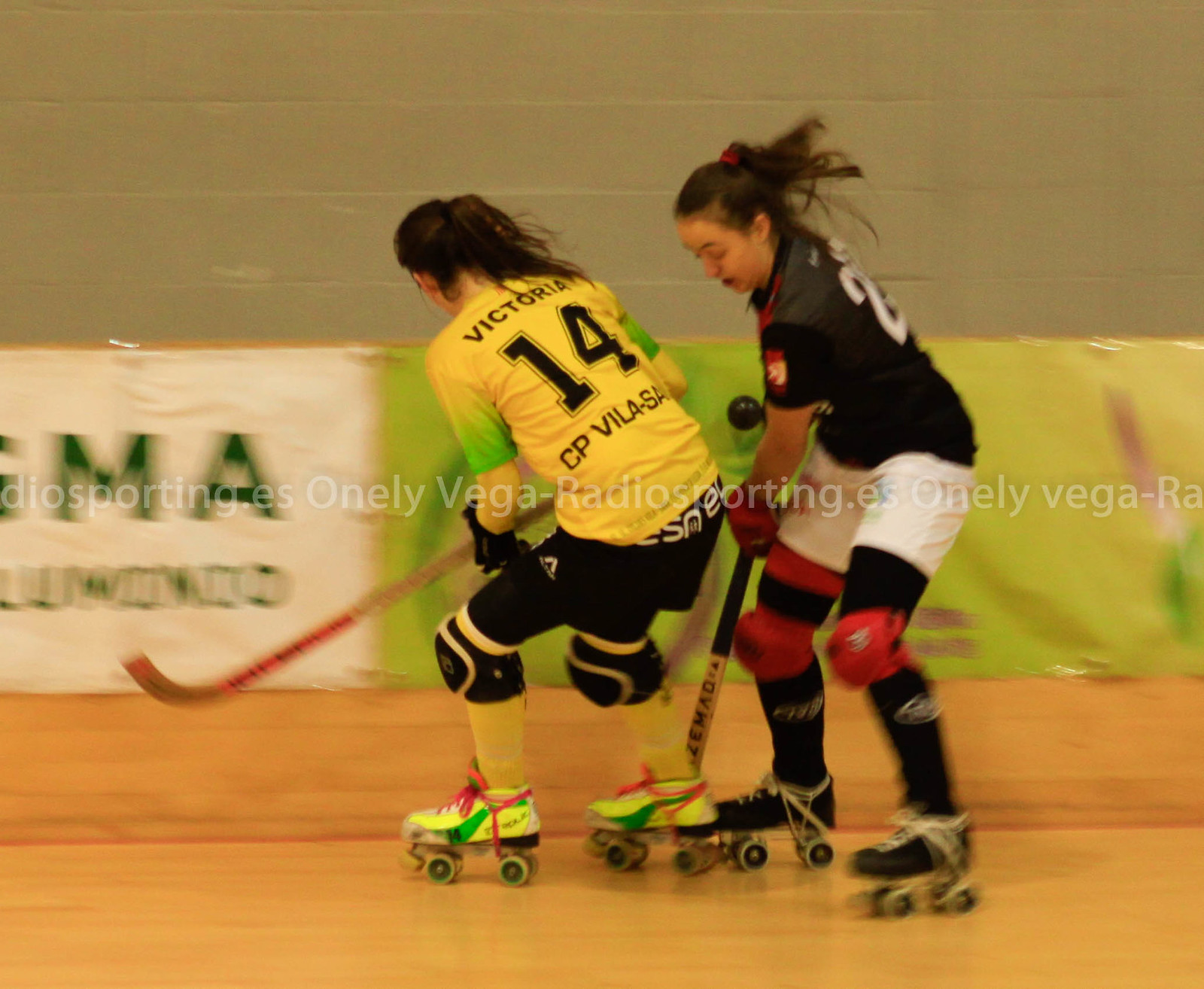In this action shot, two young women are intensely engaged in an indoor roller hockey game on a light wooden rink. Both are fully outfitted in team gear, reflecting their commitment to their sport. The woman on the left, identifiable by her yellow jersey with "VICTORIA" and the number 14, is paired with black shorts, black knee pads, yellow socks, and multicolored skates adorned with red shoelaces. She has her head turned slightly towards the back wall, her focus unwavering. In contrast, her opponent to the right wears a sleek black jersey displaying the number 2, white shorts, black stockings, and red knee pads, complete with black skates. Her dark hair flows behind her as she holds her hockey stick straight down, concentrating on the play. The background features a light gray cinder block wall, partially obscured by a faint repetitive text in white that reads "only vega-radios-reporting.es." A white and green banner hangs unfocused behind this dynamic scene, capturing the high-energy moment as the two athletes maneuver on their skates, drawing the viewer into their spirited competition.